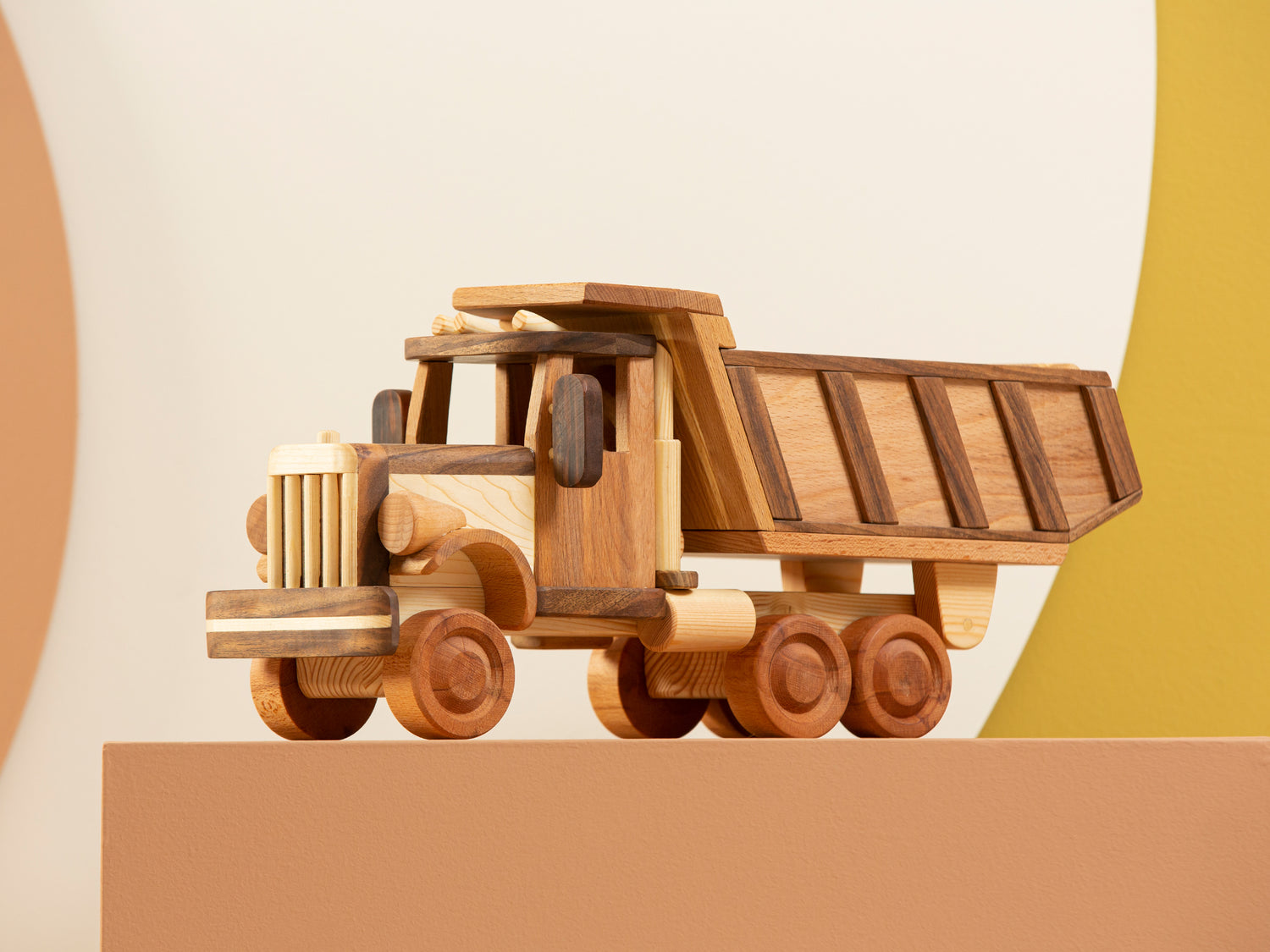The image displays a detailed indoor photograph likely intended for display or sale. In the foreground, set on a beige or light peach-colored counter or block, stands a meticulously crafted wooden dump truck. The truck features a combination of different colored woods: darker tones highlight the lines and accents of the dump area at the back, the top of the truck, the rearview mirrors, and the wheels, while lighter woods fill in the spaces between these accents. The truck's detailed formation includes a front passenger compartment and a flatbed with an open-top dump container. The background of the image is primarily white, with a mustard yellow curved shape accentuating the right side and a hint of another beige circle towards the left, adding layers and dimension to the composition.